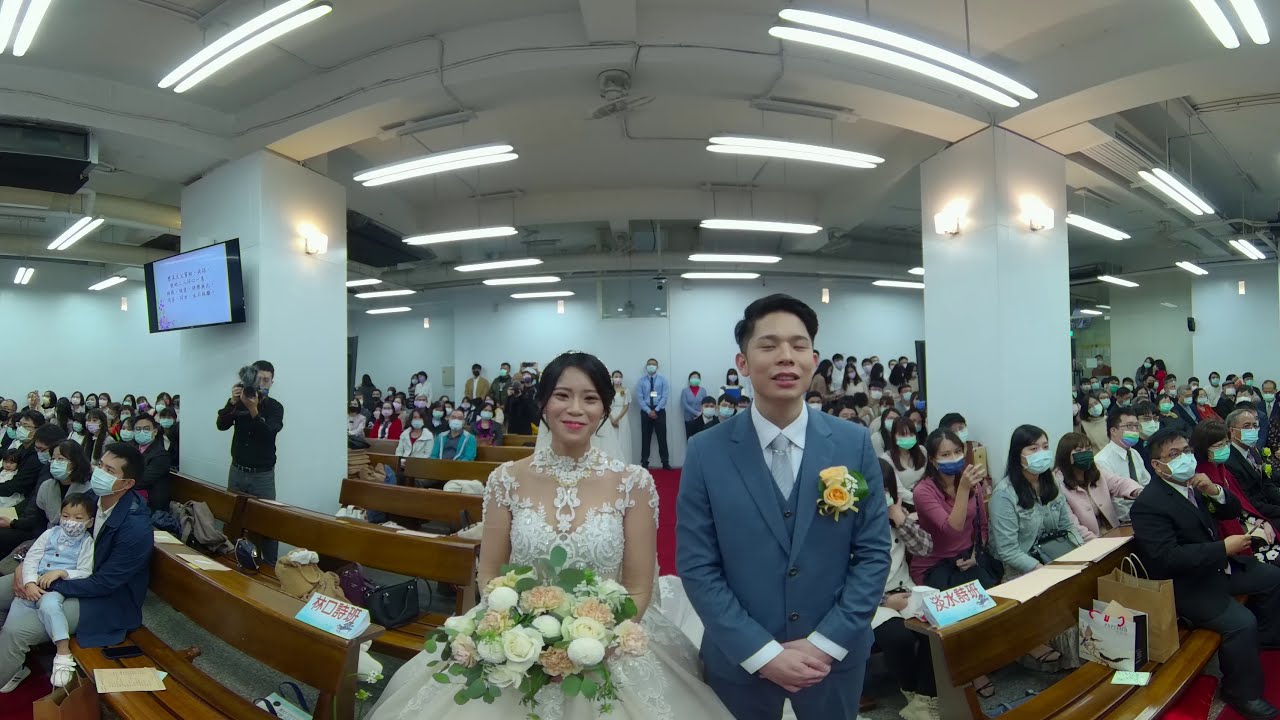The photograph captures a touching moment of a young couple’s wedding ceremony. The bride, dressed in a delicate, lace white wedding gown, is holding a large bouquet of cream, white, and light pink flowers. The groom, looking dapper in a medium blue tuxedo adorned with a yellow flower, stands by her side. Their youthful appearance and black hair indicate they might be in their late 20s.

Surrounding them is a large crowd of friends and family, all donning N95 and blue face masks, seated on wooden benches or pews. This setting, possibly a spacious courthouse or church-like venue, features bright ceiling lights illuminating the couple and the guests. A photographer dressed in black can be seen to the left, capturing the special moments. The room’s interior is characterized by white and gray walls with beams and a large TV situated against one. The overall atmosphere is one of joy, anticipation, and solemnity as the couple shares this significant milestone amidst their loved ones.